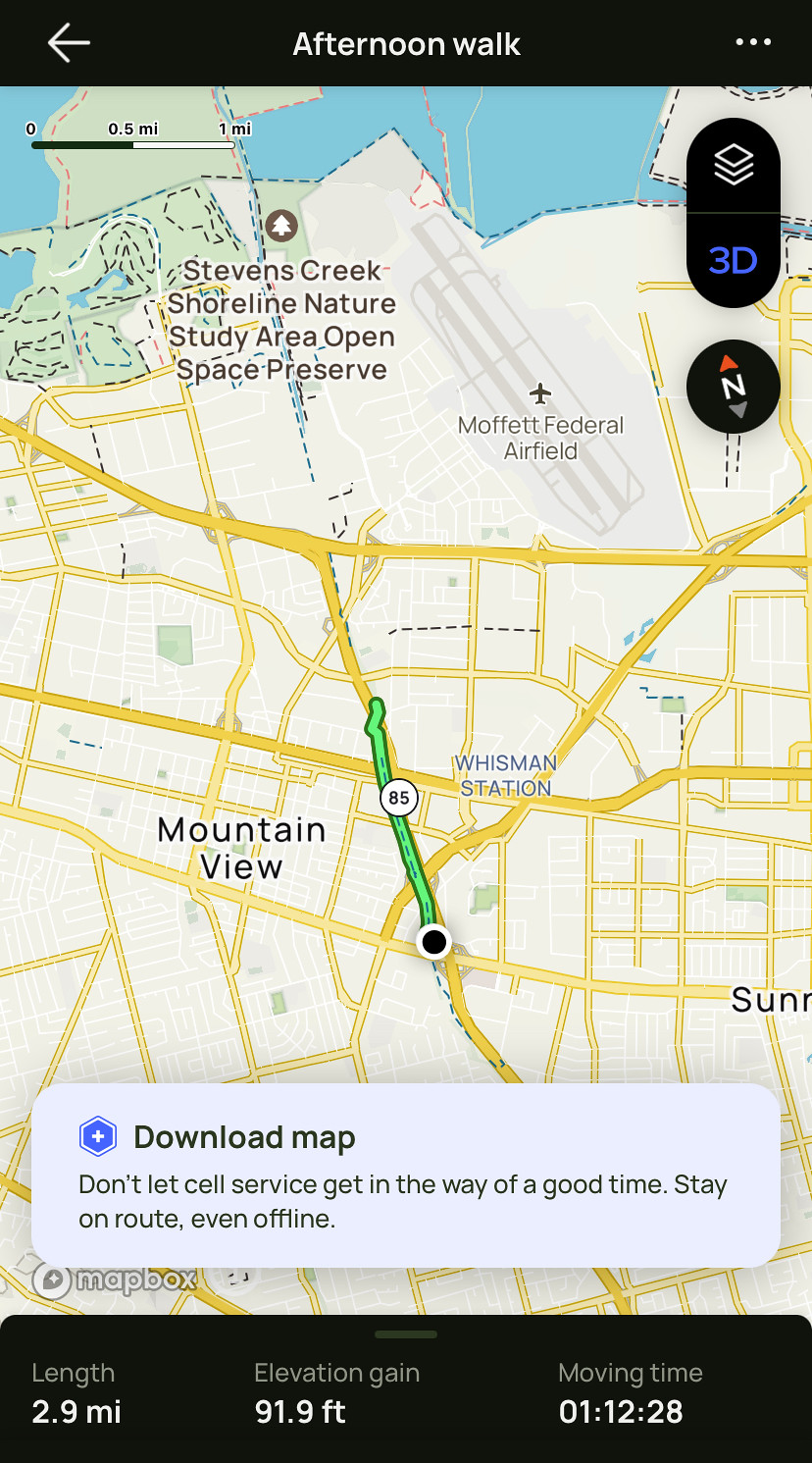This color image appears to be a screenshot from a smartphone displaying a detailed map. Across the top of the screen, there is a black bar with a white, left-facing arrow. Superimposed on the black bar is the caption "Afternoon Walk" in white text. Below this, the map showcases the "Stevens Creek Shoreline Nature Study Open Area Space Preserve."

Key areas marked on the map include "Moffett Federal Airfield" and "Wisman Station" (spelled out as W-H-I-S-M-A-N), with "Mountain View" also identified. The map features a beige background with roads illustrated in yellow and white lines, and a specific section of the yellow road highlighted in green, labeled "85."

The bottom of the image contains a white banner with black text encouraging users to "Download Map" and advising, "Don't let cell service get in the way of a good time, stay on route, even offline." Below this advisory is a black banner providing additional details in white text: "Length 2.9 miles, Elevation Gain 91.9 feet, Moving Time 1 hour 12 minutes and 28 seconds."